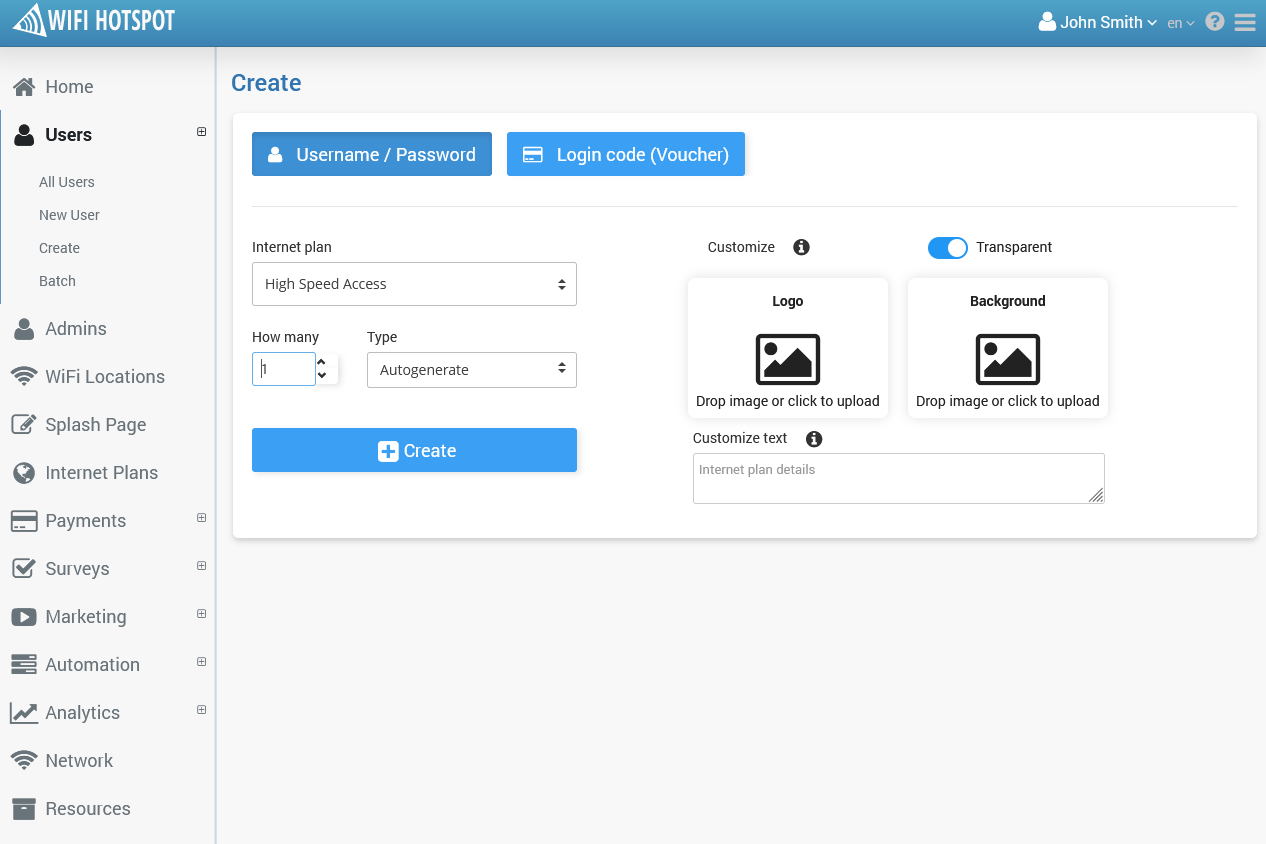- **Screenshot of Wi-Fi Hotspot Settings Interface**

The image displays the settings interface for configuring a Wi-Fi hotspot. At the very top, there is a blue banner featuring the text "Wi-Fi Hotspot" in white, accompanied by a triangular icon with a blue Wi-Fi symbol pointing to the right. In the top right corner, the account name "John Smith" is displayed next to a white icon depicting a person. Adjacent to the account name are two more icons: a three horizontal line menu drop-down and a question mark for help.

The left side of the screen features a navigation menu with the following options: Home, Users, Admins, Wi-Fi Location, Splash Page, Internet Plans, Payment, Surveys, Marketing, Automation, Analytics, Network, and Resources. The "Users" section is currently chosen, with "Create" being the active sub-menu option.

The main content area is dominated by a titled header "Create" in blue. Below this header, a white box contains further settings. At the top of this box are two blue buttons with white text: "Username/Password" and "Login Code (Voucher)." 

Next, there is a section labeled "Internet Plan" with a drop-down menu showing "High-Speed Access" as the selected option. Below this, two additional drop-down menus are present. The first, labeled "How Many," has "1" selected, while the second, labeled "Type," shows "Auto Generate" as the selected option.

Further down, a blue button with white text reading "Create" is present. This button features a plus sign inside a white box adjacent to it.

Towards the bottom of the interface, there are options for customization. There are two toggle switches labeled "Customize Transparent," with the relevant switch set to "On." Below this, there are two boxes labeled "Logo" and "Background," both of which have options for dropping or uploading an image. 

Lastly, the section titled "Customize Text" features a text box allowing users to input custom text.